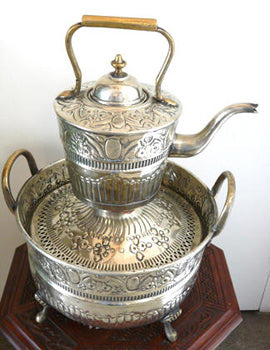The image features a vintage silver teapot intricately placed on top of a matching silver bowl, likely part of a set. The teapot boasts an elegant, elongated silver spout and a lid topped with a golden knob, accented by a wooden handle. The teapot itself is adorned with delicate etched markings in the silver, adding to its antique charm. Below, the silver bowl exhibits two brassy handles and stands on small silver legs, enhancing its sophisticated appearance. This entire arrangement sits atop a dark cherry wood side table, providing a rich contrast that highlights the silverware's vintage elegance and unified design.